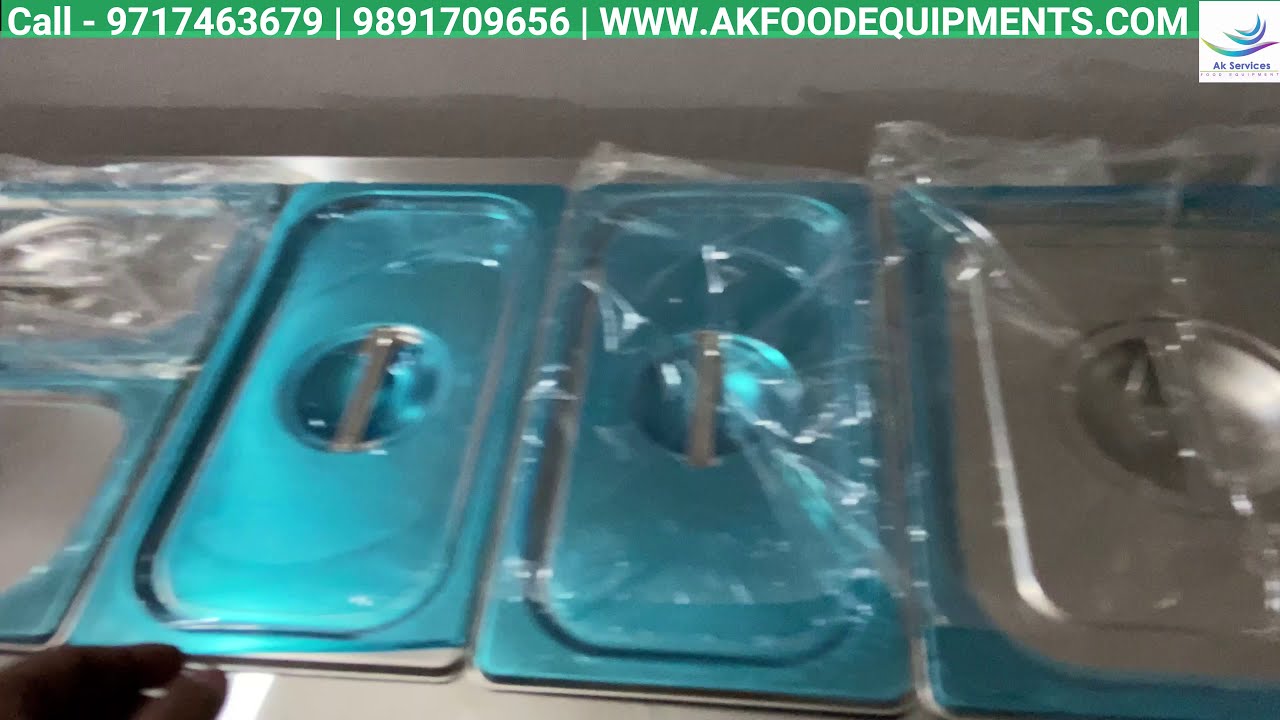This image features an assortment of new restaurant equipment, specifically metal food trays with lids, typically used in catering or buffet setups. Positioned horizontally and somewhat blurry, the photo reveals the trays wrapped in protective plastic, indicating their brand-new condition. At the forefront, a variety of lids are visible: silver lids with silver handles, two blue lids centered in the image, and an additional larger silver lid with a blue border on the right side. The trays themselves are arranged similarly to how they would be displayed in a buffet setting, with rectangular and square shapes. The top of the image displays a green banner featuring contact information in white text: "Call 971-746-3679 | 989-170-9656 | www.akfoodequipments.com." Additionally, the upper right-hand corner showcases a small white square logo containing blue swirls and the text "AK Services." The overall presentation suggests that this might be a still from a low-resolution YouTube product video, aimed at advertising these catering equipment pieces.